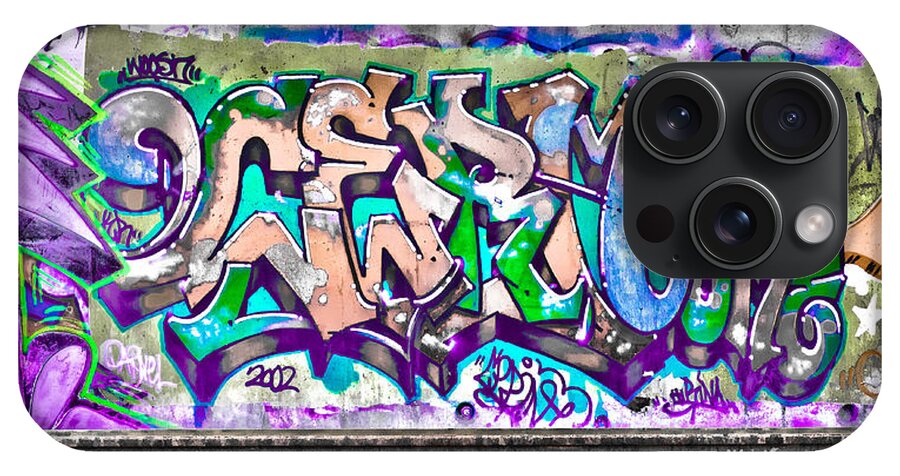The image depicts the back of an iPhone, identifiable by its distinctive three-camera setup arranged in a black square in the upper right-hand corner, with two cameras on top, one below them in the center, a white dot to the right, and a black dot to the left. The phone is oriented in landscape mode, with the shorter sides at the top and bottom. The iPhone is sheathed in a vibrant graffiti-style case, adorned with a collision of colors including purples, greens, peaches, blues, oranges, and whites. The graffiti features bubbly and stylized writing, typical of such art, with no clear, readable letters or words, though some numbers "2002" can be discerned. The chaotic yet captivating design of the case contrasts with the dark color of the iPhone itself. The image is clear and brightly lit, highlighting the bold and dynamic artwork on the phone case.